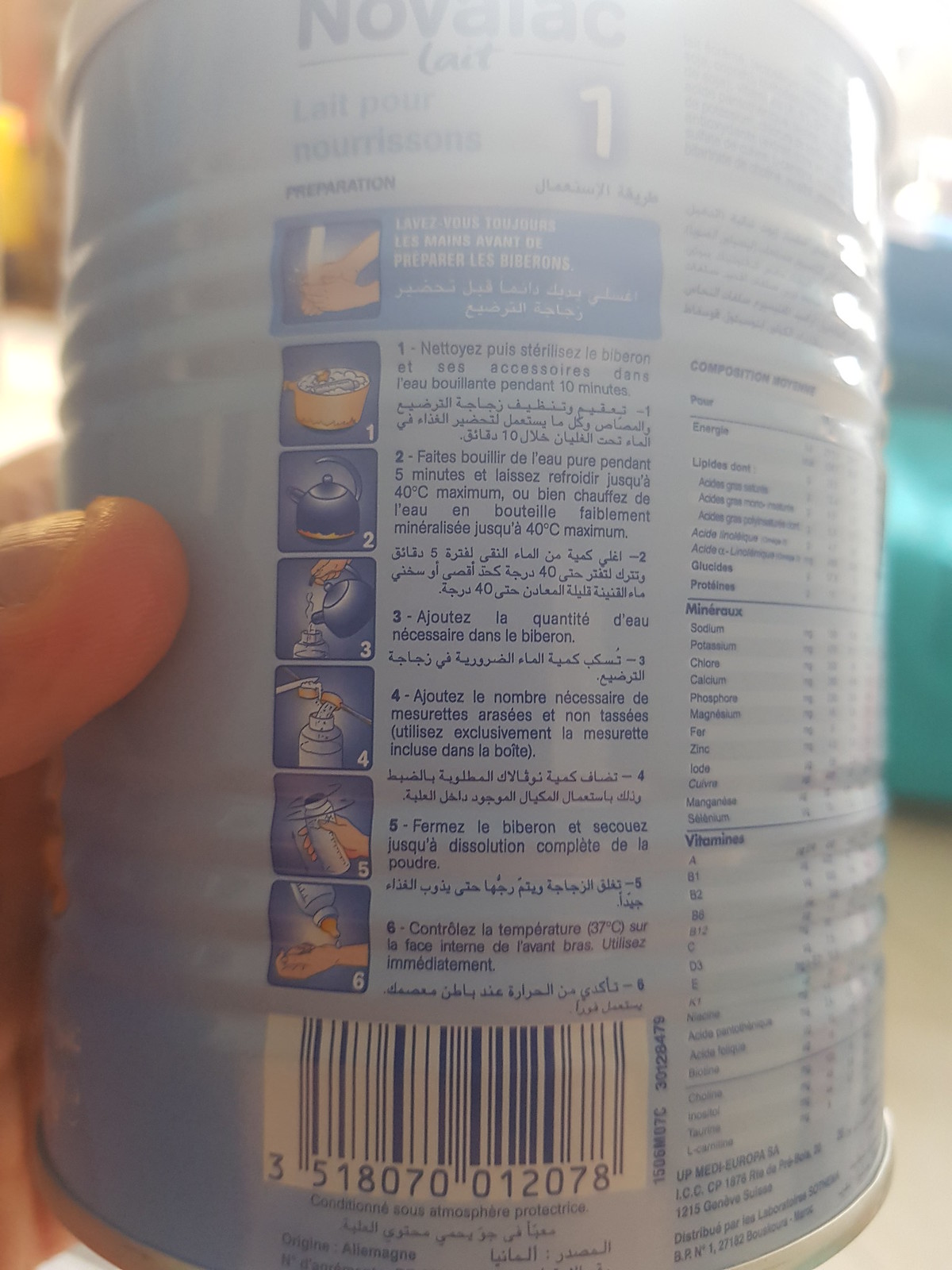This image is a colour photograph taken in portrait orientation, featuring an extreme close-up of a metallic food tin with undulating ribbed sections at the bottom third and top third of its circumference. The tin, held upright by someone's left hand, reveals a horizontally aligned barcode at the bottom, marked with the numbers "3 518070 012078." Above the barcode, there are six illustrated, vertically arranged coloured images depicting a step-by-step usage guide, which includes washing hands, boiling the contents, shaking the tin, transferring it into a bottle, and testing the temperature on the back of the wrist before feeding—a process indicative of preparing baby formula. Although the text on the tin is in a foreign language, possibly a Romance language like French, the detailed illustrations effectively communicate the necessary steps. The backdrop features a linoleum floor and a teal green seat, slightly out of focus and highlighting the can's light blue colour.